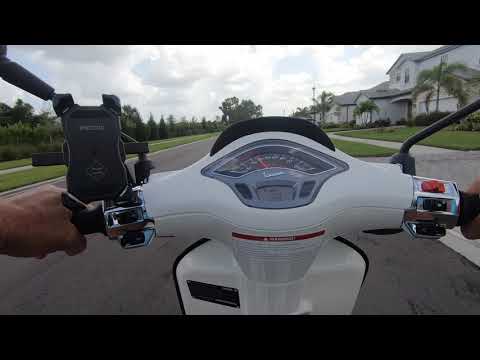In this vibrant, first-person perspective shot, we see an individual riding a white moped down an unmarked, light gray asphalt road in a serene residential neighborhood. The moped's handlebar and speedometer, mounted with a phone or GPS holder on the left, are centered prominently in the image. On both sides of the road are well-manicured grass sections leading to sidewalks. To the left, a sidewalk is bordered by more grass and a row of trees, while on the right, the sidewalk runs past front lawns of sizable two-story houses with gray roofs and pristine white walls, each boasting a palm tree in its front yard. Above, patches of sky filled with clouds complete the picturesque, upper-class suburban setting, suggesting a pleasant day outdoors.